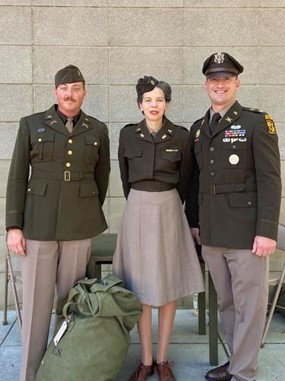The photograph depicts three members of the military standing in front of a smoothly textured light gray stone brick wall. In the background, behind them, there is a table that appears to be either gray or dark green. Positioned between the individuals in the front of the image is a bag tied up with a white label, though the label is not clearly visible from the camera's angle.

At the center of the photo stands a Caucasian woman, aged between 40 to 50 years, dressed in a military uniform consisting of a dark grayish-green long-sleeve top and a gray skirt that reaches her knees. She is wearing brown shoes and a hat, with some pins around her collar.

Flanking her on either side are two Caucasian men. The man on the left, aged between 30 to 40 years old, sports a mustache and is dressed in a similar dark green military jacket with three buttons, gray dress pants, and a cap. He also has several pins around his collar.

The man on the right, who appears to be the youngest, also between 30 to 40 years old, is dressed in the same dark green military jacket, gray dress pants, and a cap. His jacket features several pins and a medal, as well as a ranking insignia. Unlike the other two, he is wearing a tie and is smiling with his teeth showing.